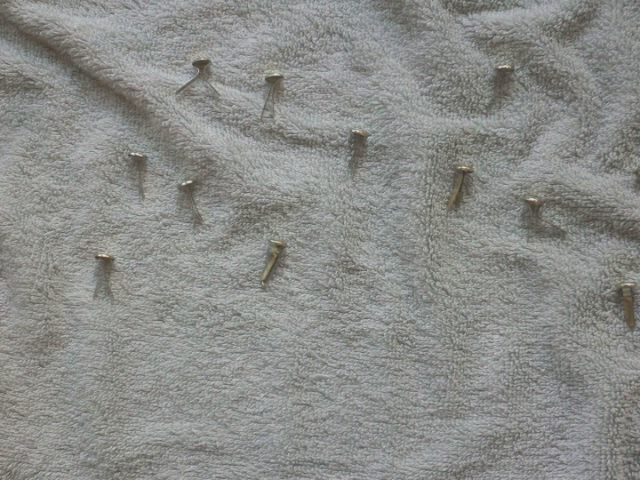On a soft, slightly crinkled, light gray surface—likely a towel or a blanket—lies a scattered arrangement of silver nails. The nails, reminiscent of thumbtacks with their two metal pieces that spread apart, are placed in a somewhat haphazard manner. In one area, a slanted row of six nails descends from the upper left to the lower right. In the top right corner rests a single nail, and another solitary nail can be found on the top left. Toward the middle left, a group of three nails appears, with some leaning to the right. On the bottom left, a nail's shadow is visible, though it seems the bottom part is missing. Finally, in the lower middle, another nail leans slightly to the right, and the last nail is positioned in the bottom right-hand corner.